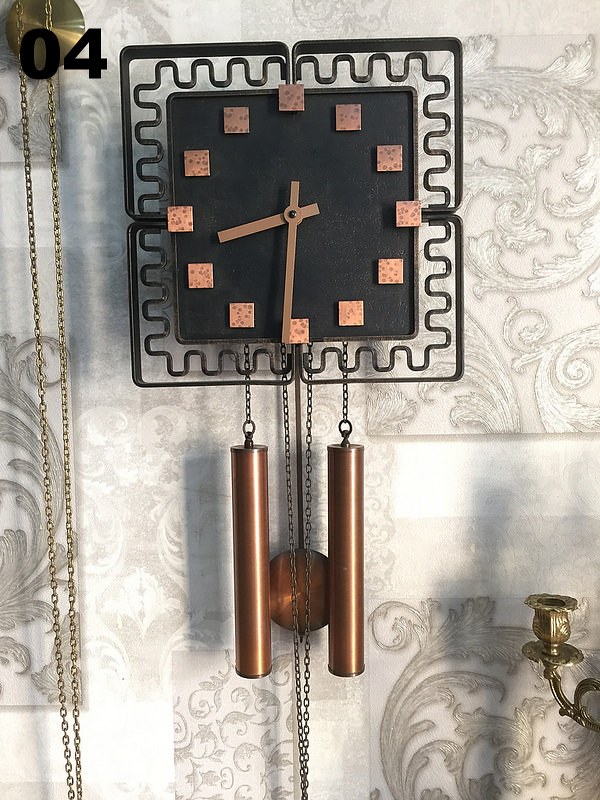This photograph features a stylish, square-shaped clock that exudes a mix of modern and vintage aesthetics. The clock is predominantly black with distinct copper accents, highlighting its intricate design. Made from metal, it boasts a sturdy square metal frame adorned with twisting metal decorations that run its length, adding a touch of elegance to its robust structure.

The clock face, also square, is uniquely designed with smaller copper square shapes affixed to it, representing the hours without traditional numerals. The two copper hands elegantly point to the time, and notably, there is no second hand. Attached to the clock are copper-colored rods and a pendulum, which gently swings back and forth with each passing second, adding a dynamic element to the otherwise static timepiece.

This eye-catching clock is mounted on a wall adorned with ornate wallpaper. The wallpaper features a sophisticated pattern of squares filled with intricate floral designs and swirling motifs in gold and white, providing a luxuriant backdrop that complements the clock’s aesthetic.